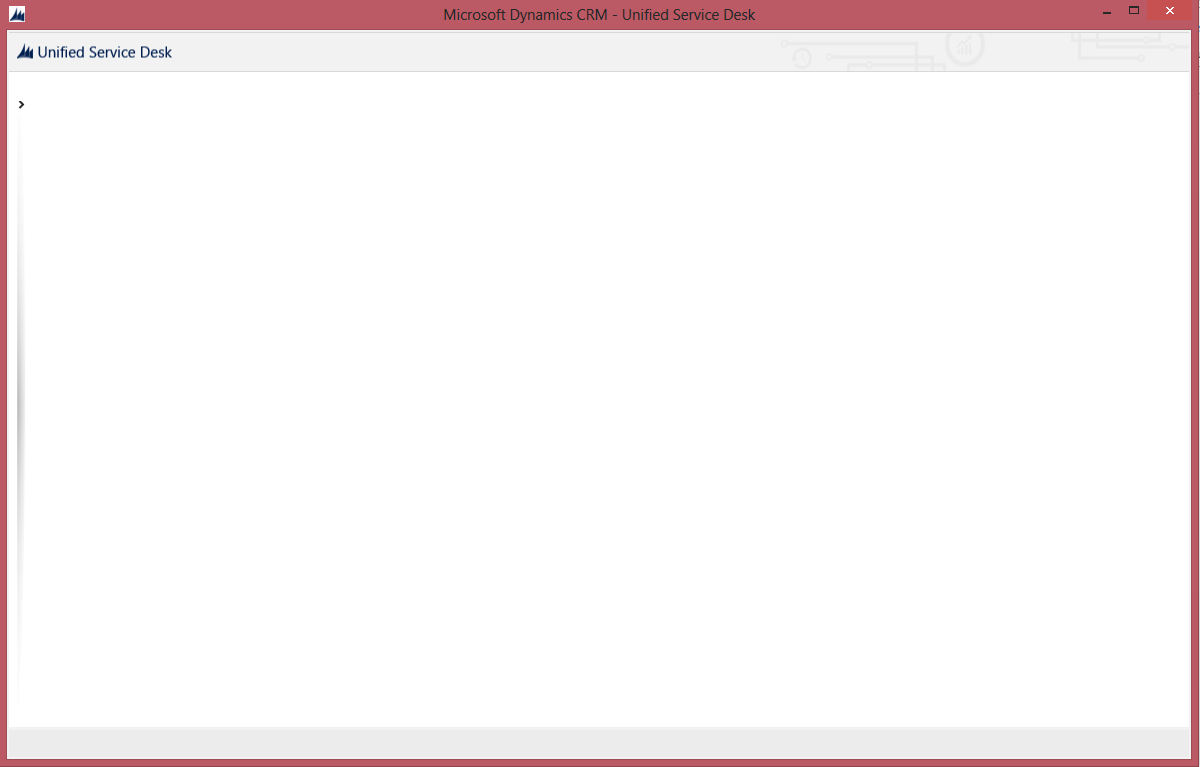The image showcases a web page that appears to be blank, possibly indicating it hasn't loaded correctly, due to an error, or it cannot load at all. The page is enclosed by a red border, featuring a distinctive red header. At the top, written in a small black font, is the text "Microsoft Dynamics CRM, Unified Service Desk." On the right side of the header are the typical icons for closing the screen, expanding it, or minimizing the tab. On the far left of the header, a logo resembling three somewhat misshapen triangles or peaks is displayed, next to which the text "Unified Service Desk" is written. The main body of the web page is entirely white, devoid of any content or elements, presenting a stark and empty landing page.